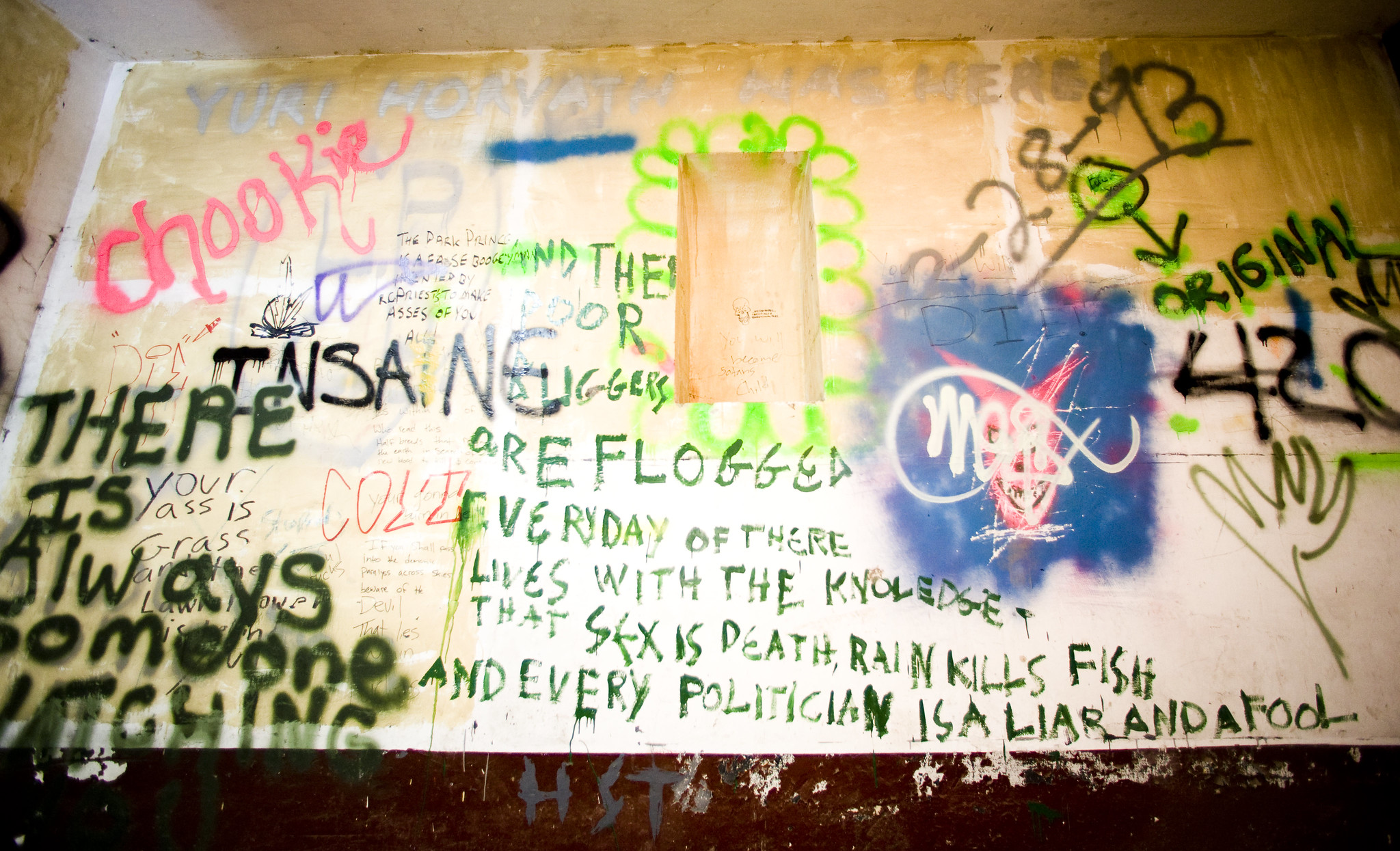This photograph showcases an interior wall, likely within an abandoned building, that's entirely covered in chaotic graffiti. The once predominantly white wall now displays patches of mottled yellowish-orange and blue paint, adding to the visual cacophony. Various texts, tags, and designs in multiple colors and writing styles dominate the wall, creating a vibrant yet messy collage.

In the upper left corner, the word "Chuki" (alternatively spelled "Chewky" and "Chuki" in pink letters) is prominently displayed. Nearby, messages such as "there is always someone watching" are visible, written in green paint at the lower left. The central part of the image contains a lengthy, cryptic message in green letters, stating, "the poor are flogged every day of their lives with the knowledge that sex is death, rain kills fish, and every politician is a liar and a fool." 

Additionally, to the right-hand side, the phrase "Original 42" (also read as "original 420" with an arrow pointing down) can be seen alongside some barely legible tags and messages. There are also other elements including a gray "HST" on a worn, possibly rusted red area positioned at the very bottom. The graffiti spans a variety of colors including pink, green, blue, black, and yellow, contributing to the overall sense of disorder and neglect.